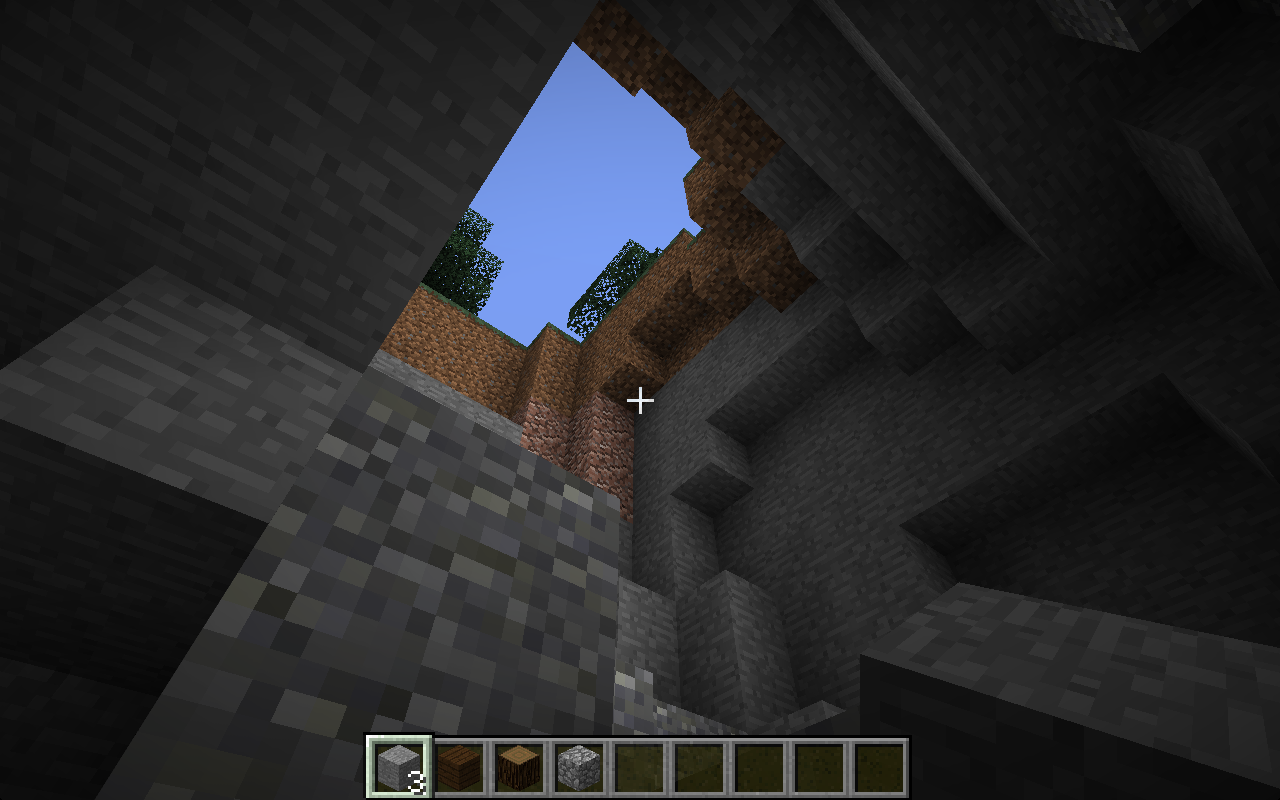In this detailed Minecraft screen grab, we are positioned at the bottom of a dark, cavernous structure, peering upwards through a roughly carved opening. The structure features haphazardly arranged gray stone and dirt block walls, reminiscent of an Escher-esque construction with walls jutting out at various angles, giving it a chaotic, jumbled appearance. Centered above, there is a visible break in the ceiling through which a patch of blue daytime sky can be seen, bordered by greenery and hints of tree tops. The distinct pixelated aesthetic of Minecraft is evident throughout the image. At the base of the screen, a menu bar displays various types of blocks available for building, emphasizing the typical in-game interface.